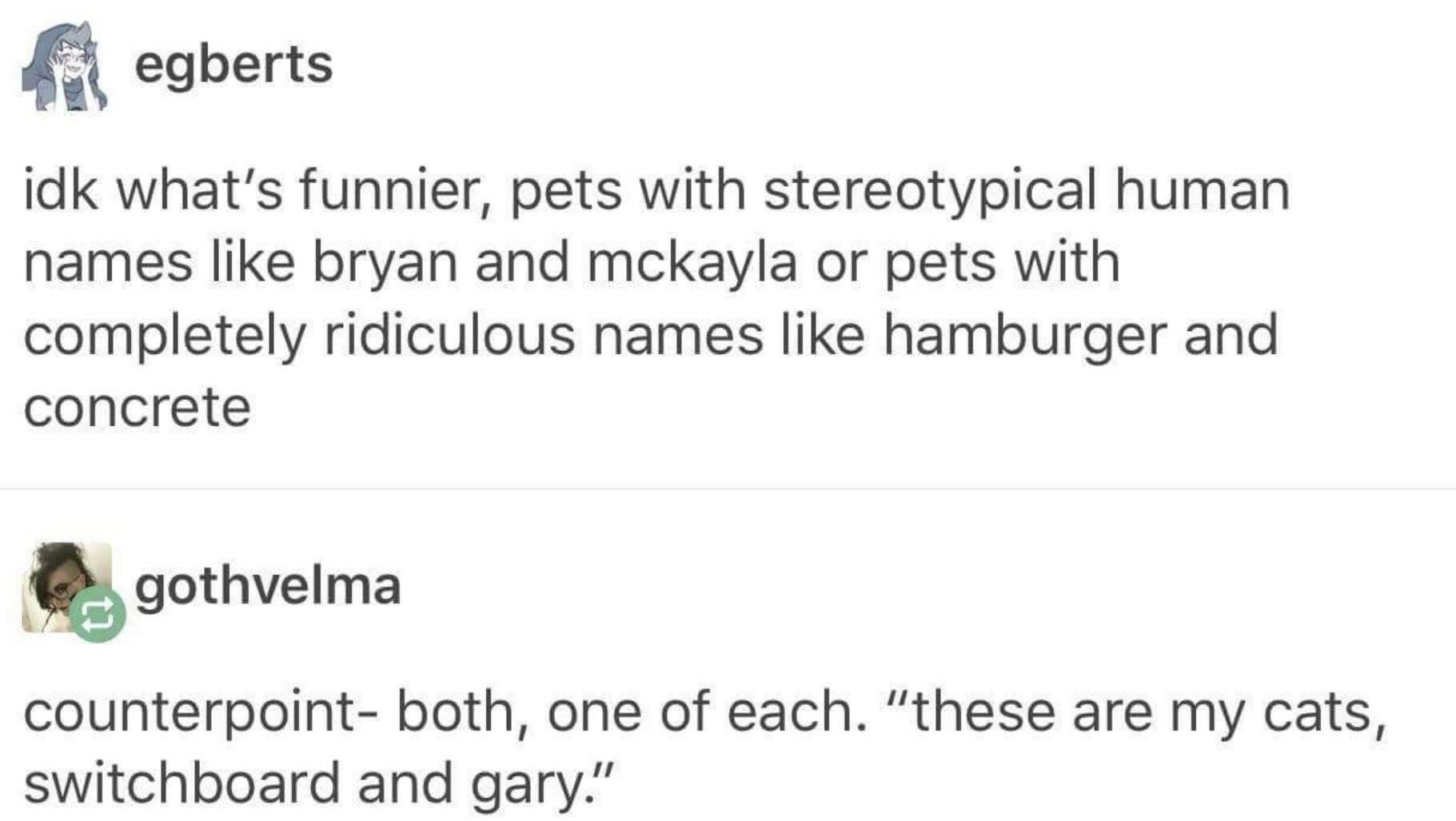This image is a screenshot of a conversation on a social media platform, likely Tumblr, featuring a post by Egberts and a reply by Gothelma. Egberts' post includes a small cartoon character of a girl with grey spiky hair and blush on her cheeks, wearing a dark blue hood and scarf. The text in Egberts' post reads: "IDK what's funnier, pets with stereotypical human names like Brian or McKayla, or pets with completely ridiculous names like Hamburger and Concrete." Gothelma responds to this with a comment, indicated by a green border around their profile picture of the horror character Chucky, and says: "Counterpoint—both, one of each. These are my cats, Switchboard and Gary." The reply is marked by an arrow pointing to the right, and another arrow pointing back to the left, signaling the back-and-forth nature of the conversation.